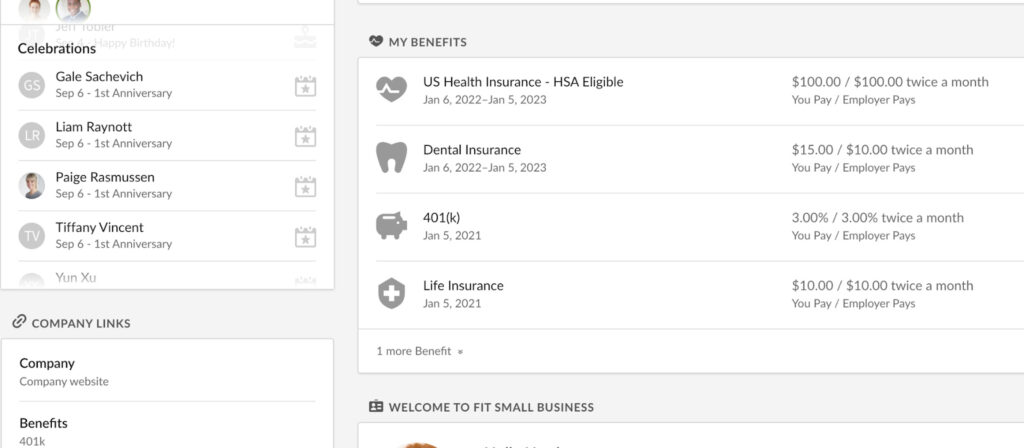**Detailed Descriptive Caption**

This screenshot comprises multiple sections, predominantly featuring white and gray tones. On the left side, two circular icons display images of a light-skinned person and a darker-skinned person. Centered above these icons in black text is the word "Celebrations."

Below this title, a series of detailed entries are listed, each marked with a calendar icon. The entries begin with:

- GS (Gail Samvich), September 6th, for a first anniversary.
- L.R. (Liam Reinott), September 6th, for a first anniversary.
- Paige Ramson, September 6th, for a first anniversary, along with an image of a light-skinned woman.
- Tiffany Vincent, September 6th, for a first anniversary, accompanied by a TV icon.
- YUNXU is also listed, with the name prominently presented within a gray circle.

Further down, there is a section titled "Company Links" with a paper clip icon beside it, followed by two white boxes separated by a thin gray line:
- The first box contains links labeled as "Company" and "Company Website."
- The second box lists "Benefits" and "401k."

To the right, a thin gray box is labeled "My Benefits" with a heart and wave icon. Below it, several white boxes separated by thin gray lines list various benefits, each with corresponding icons and details:

1. **US Health Insurance** (Heart with wave icon)
   - **Coverage Period**: January 6th, 2022 to January 5th, 2023
   - **Cost**: $100 (employee) / $100 (employer) paid twice a month

2. **Dental Insurance** (Tooth icon)
   - **Coverage Period**: January 6th, 2022 to January 5th, 2023
   - **Cost**: $15 (employee) / $10 (employer) paid twice a month

3. **401k** (Piggy bank icon)
   - **Start Date**: January 5th, 2021
   - **Contribution**: 3% (employee) / 3% (employer) paid twice a month

4. **Life Insurance** (Shield with a white cross icon)
   - **Start Date**: January 5th, 2021
   - **Cost**: $10 (employee) / $10 (employer) paid twice a month

Below these entries, another box titled "One More Benefit" includes the message, "Welcome to Fit Small Business," accompanied by a small badge icon with lines and a person.

At the bottom of the screenshot, there is a visible segment of a white box partially covered by a circle.